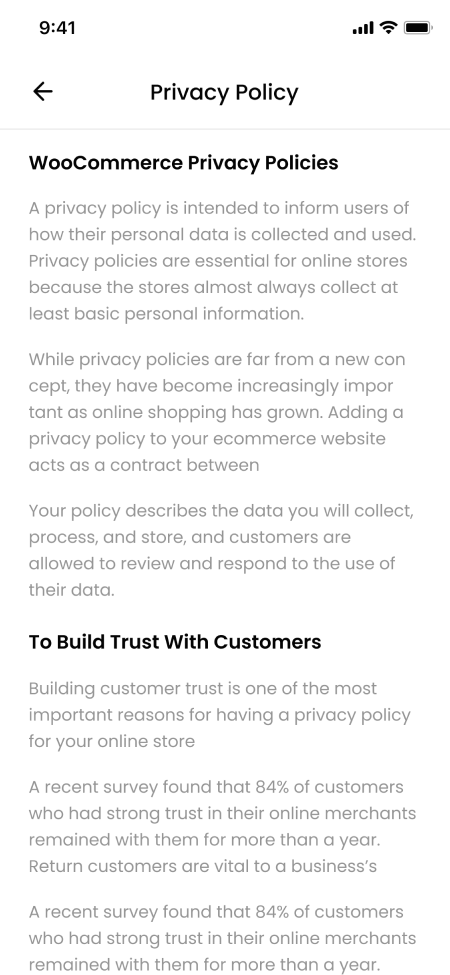The image features a white background with the text "941 Privacy Policy" accompanied by a left arrow indicating the "WooCommerce Privacy Policies." The primary focus is on the importance of privacy policies for e-commerce websites. 

A privacy policy outlines how personal data is collected, processed, and used, which is crucial for online stores that routinely gather basic personal information from customers. Despite their longstanding existence, privacy policies have gained increased significance with the rise of online shopping. 

Implementing a privacy policy on an e-commerce site serves as a contract between the business and its customers, detailing the specifics of data collection, processing, and storage. Customers are granted the opportunity to review and respond to the usage of their data, thereby fostering transparency and trust. 

Building customer trust is a key reason for maintaining a privacy policy for online stores. According to a recent survey, 84% of customers who had strong trust in their online merchants continued to shop with them for over a year. 

In summary, the image emphasizes the critical role of privacy policies in protecting customer data and maintaining long-term trust between online merchants and their customers.